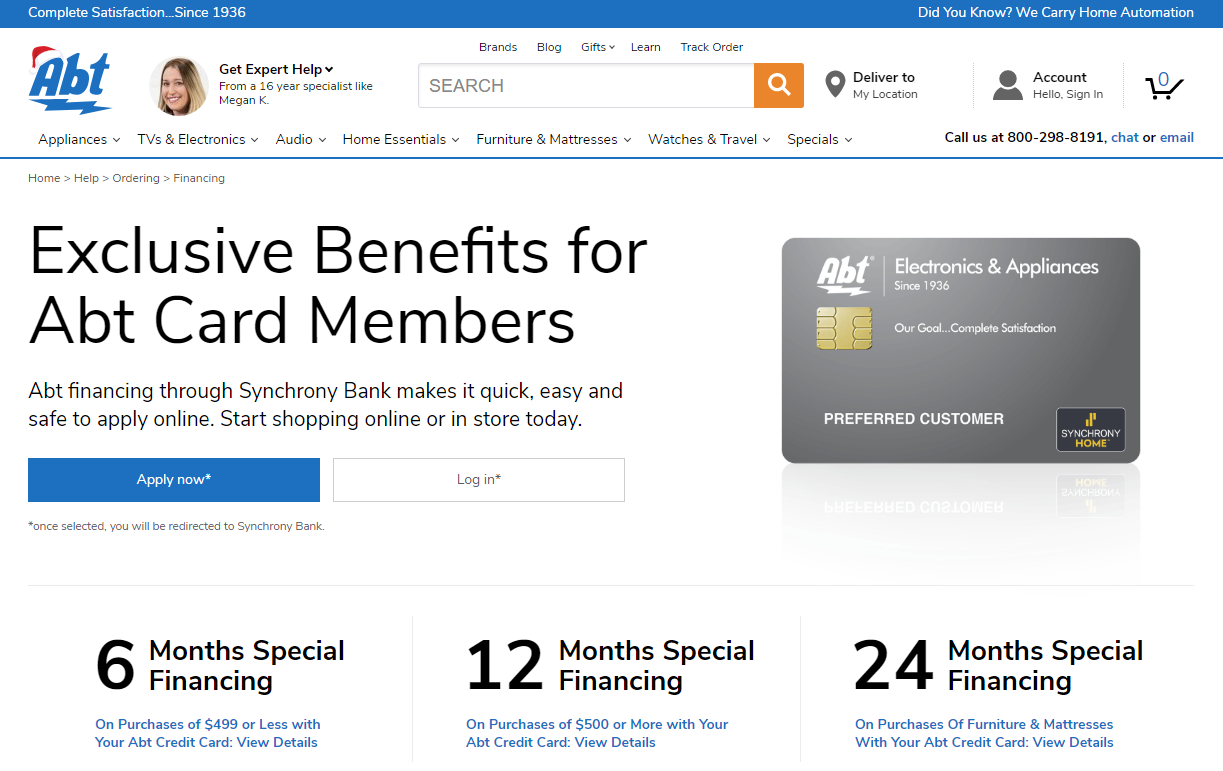The screenshot depicts an online application’s web page. At the top of the page is a long horizontal blue bar. On the left side of this blue bar is a logo reading "ABT," which is underlined by a blue lightning bolt. Positioned next to the logo is a small profile image of a smiling woman. Accompanying this profile image, the text reads, "Get expert help from a 16-year specialist like Megan Kay." Further to the right lies a search bar, and at the far right corner are icons for account sign-in and a shopping cart, which indicates there are currently zero items in the cart.

The main section of the web page features a mostly white background. On the left side of this section, prominent bold text reads, "Exclusive benefits for ABT card members."